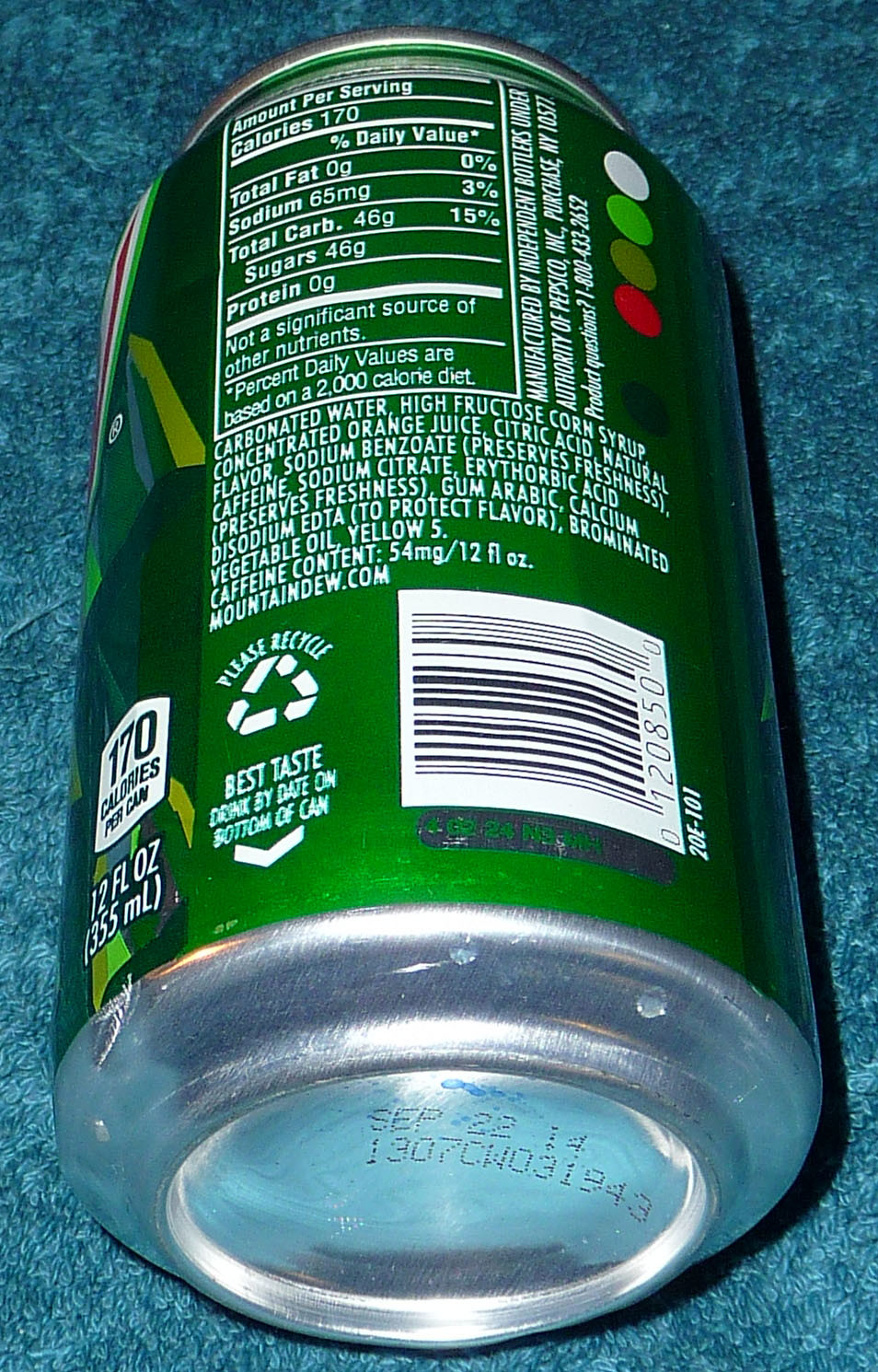The photograph captures a realistic side view of a green soda can lying on its side against a blue carpet or towel-like background. The image prominently displays the nutritional information side of the can with a detailed white nutrition label. The label includes the serving size details, stating "calories 170" per serving, alongside the percentage daily values: total fat 0g (0%), sodium 65mg (6%), total carbohydrate 46g (15%), sugars 46g, and protein 0g. The ingredients listed include carbonated water, high fructose corn syrup, concentrated orange juice, citric acid, natural flavor, sodium benzoate (preserves freshness), caffeine, sodium citrate, erythorbic acid (preserves freshness), gum arabic, calcium disodium EDTA (to protect flavor), brominated vegetable oil, and yellow 5. At the bottom of the can, it states "12 FL OZ (355 mL)" and features an expiration date of September 22, 2014.

On the right-hand side of the label are a white barcode and a note indicating the beverage is "manufactured by Independent Bottlers under the authority of PepsiCo Incorporated" with an address and a phone number. Near the bottom, the can has a "Please Recycle" message with a recycling symbol. The top right section of the can features a sequence of colored dots: white, light green, darker green, and red. Beside this, a small white square near the bottom amplifies the message, stating "170 calories per can" in dark green lettering on a white background. The combination of these details and the setup emphasizes the informative and structured design of the soda can, blending both visual and textual elements seamlessly.